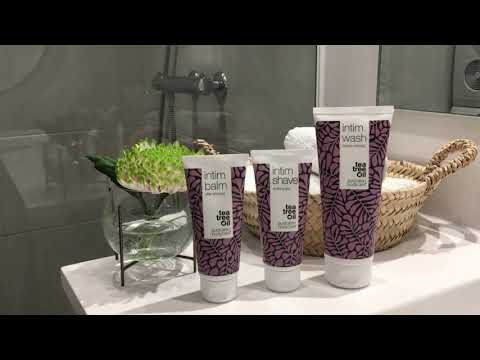The image captures a pristine white bathroom counter with a shower visible in the background, featuring glass doors and silver metal faucets. Prominently displayed on the counter are three bottles of Intim products arranged from left to right. The two smaller bottles, marked "Intim Balm" and "Intim Shave," flank a larger bottle labeled "Intim Wash." Each bottle features a distinctive design with light purple leaves set against a dark purple background, and they all mention tea tree oil. Behind these bottles, there is a clear bulb vase with a green flower on a metal stand and a light-colored, short round wicker basket containing white hand towels.